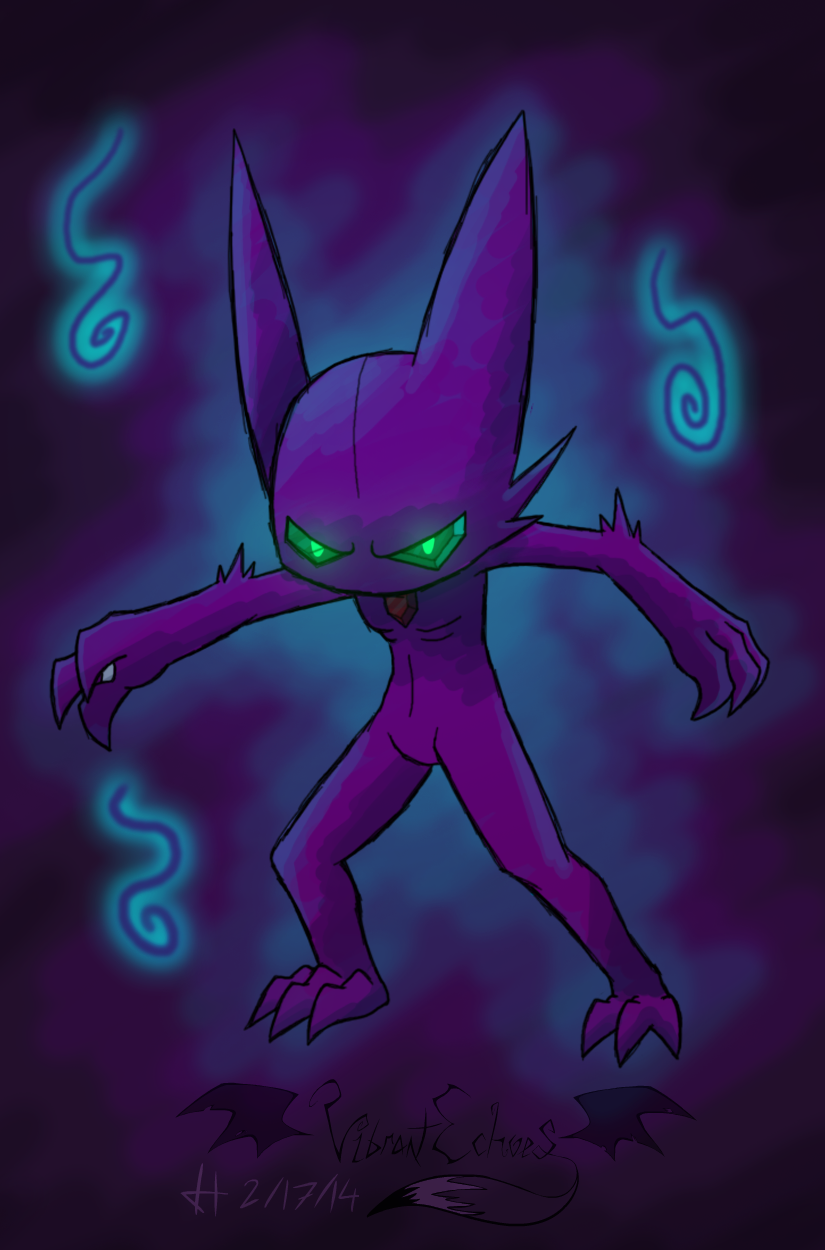The image depicts a dark purple cartoon-like character with an elongated, slender body and no visible neck. Its most striking feature is a pair of glowing, bright green eyes set in oddly shaped, almost oval sockets. The character has long, pointed ears and arms that stretch out, ending in hands with three clawed fingers on each side. Similarly, its legs are normal-sized but culminate in feet with three toes each.

The background consists of a dark purple and teal gradient, accented by vibrant, bright blue highlights that outline the character. Additionally, there are dynamic zigzag and curly Q lines in teal around the figure, adding a sense of motion and depth. Above and below the character, these lines mimic the bright blue echo effect surrounding the figure.

The chest of the character appears caved in, adorned with a mysterious piece that could be a necklace or an emerald-like accessory. The eyes differ slightly in description, with hints of being either squinty yellow or glowing green, adding to its eerie, enigmatic presence. Notably, there is an artist's signature and date, 2-17-14, at the bottom of the piece, suggesting it is a graphic art creation, possibly fan art, of a monster-like or Pokemon-inspired figure.